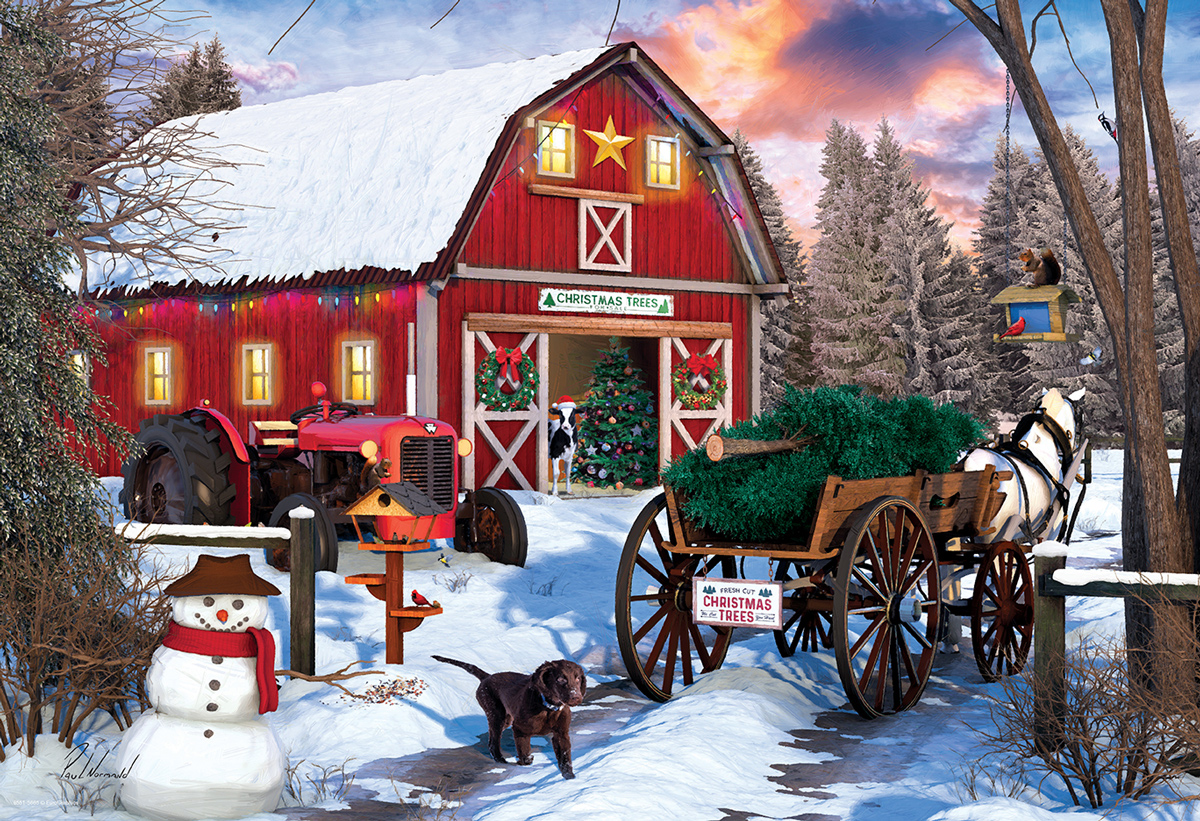In this picturesque, heavily-detailed winter scene, a red wooden shop, resembling a barn, stands prominently with a triangular snow-covered roof. This barn-like structure features a festive green sign above its open entrance that reads "Christmas Trees," adorned with a small picture of a tree. Two upper front windows emit a warm yellow glow, flanking a decorative star, while the ground level showcases Christmas wreaths with red bows. The right side of the barn has three windows, lined with Christmas lights, and one more window on the front is visible.

In the foreground, a horse-drawn carriage moves away from the viewer. The white horse pulls a green Christmas tree loaded onto the wagon, and a black dog follows behind. Nearby, on the bottom left corner, stands a cheerful snowman sporting a brown hat and a red scarf. A striking red tractor with large back wheels is parked to the side of the shop.

The setting is framed by a backdrop of tall, snow-draped evergreen pine trees. Above, the sky features a gradient of blue, orange, and purple hues with wispy clouds. Adding to the festive touch, a bird feeder hanging from a bare tree branches overhead, attracting a vibrant red cardinal. The packed snow on the ground reveals patches of worn earth where the carriage has trekked.